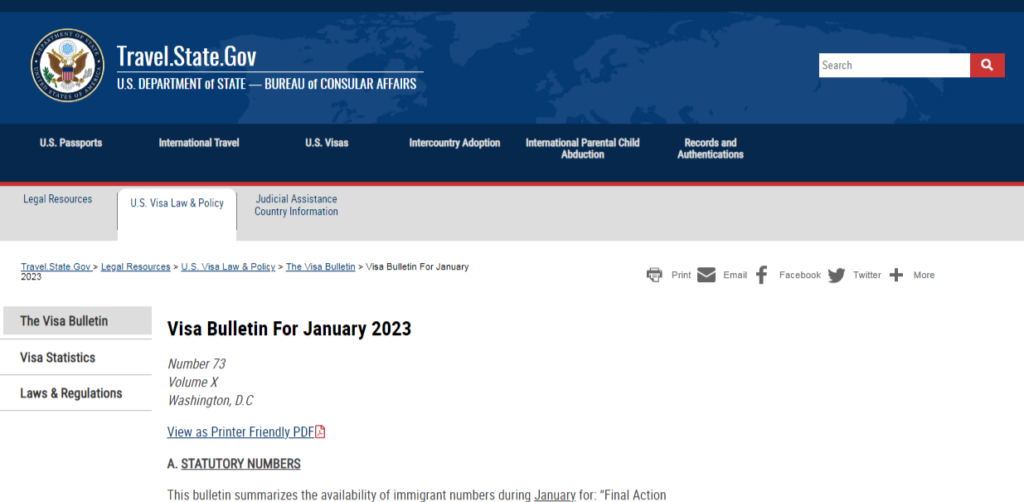This image is a detailed screenshot from the official government website, travel.state.gov. The top of the page features a prominent blue header, subtly adorned with a topographical map design embedded as a backdrop. In the upper left-hand corner of this header, the official government seal is displayed, showcasing eagle wings and a shield, signifying the authority and authenticity of the site.

To the right of the seal, white text reads "travel.state.gov," followed by a description: "U.S. Department of State Bureau of Consular Affairs." Directly below the header, a darker blue navigation bar spans horizontally across the screen, listing various critical areas of interest in white text. This navigation bar includes clickable options for "U.S. Passports," "International Travel," "U.S. Visas," "Inter-country Adoption," "International Parental Child Abduction," and "Records and Authentication."

Beneath this main navigation bar, there are three additional tabs offering more specific resources: "Legal Resources," "U.S. Visa Law and Policy," and "Judicial Assistance Country Information." The screenshot highlights the middle tab, "U.S. Visa Law and Policy," indicating that it has been selected. Subsequently, the section below displays the title "Visa Bulletin for January 2023," along with a downloadable link to a PDF file containing the bulletin. This detailed layout and clear navigation illustrate the website’s comprehensive approach to providing vital travel and visa-related information to users.